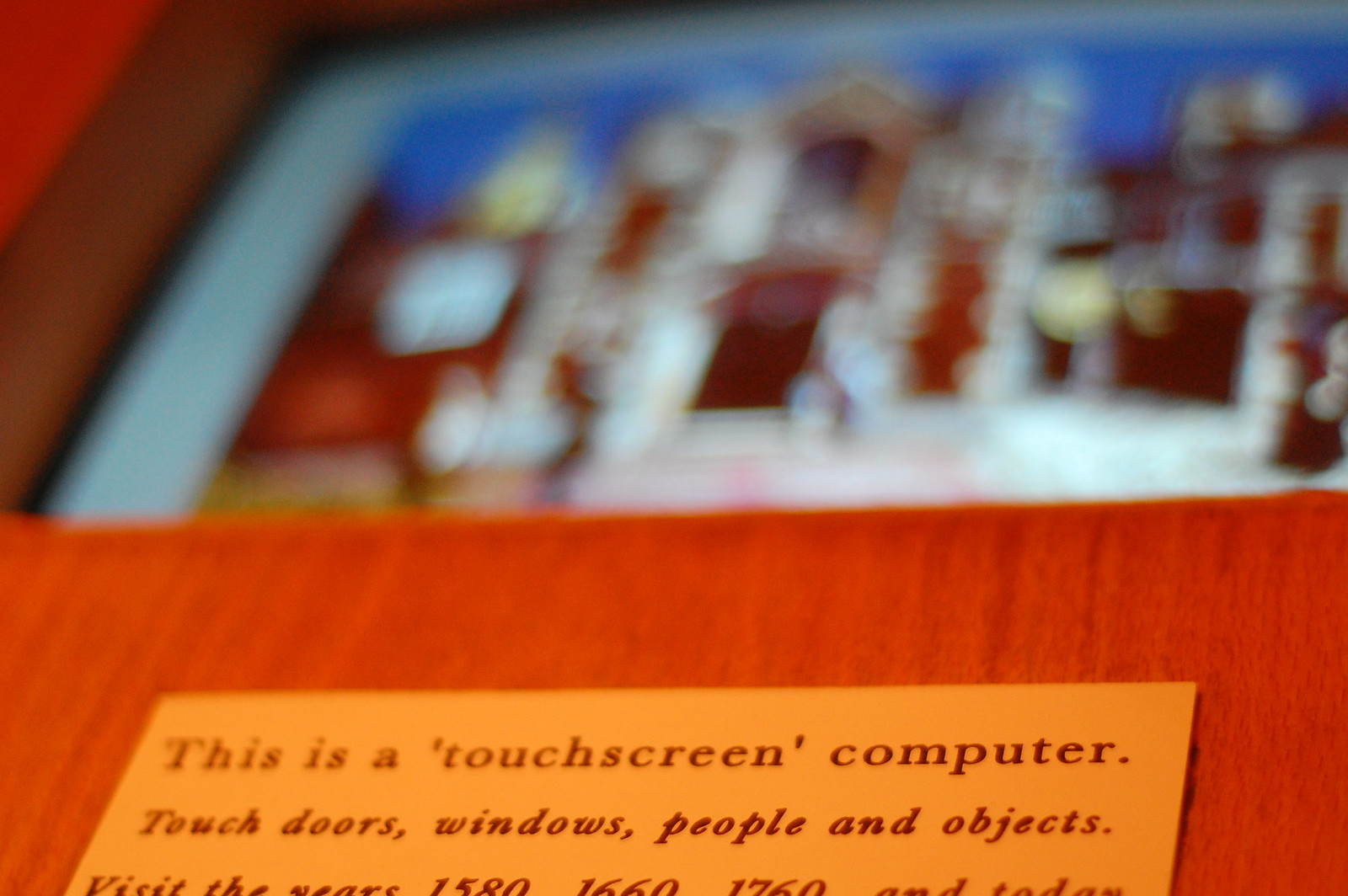The image features a wide rectangular view of a label situated beneath a partially visible picture, composed on a reddish-orange fabric-like background running horizontally across the bottom portion. Prominently placed halfway down this section is a yellow note card, broader than it is tall and slightly cut off at the bottom edge of the image. The note card displays black lettering stating, "This is a 'touchscreen computer'." Beneath this, in italicized text, it reads, "Touch doors, windows, people, and objects." Following this, the note instructs viewers to "visit the years 1580, 1660, 1760, and today." The upper portion of the image shows a blurry screen with hints of red and white, adding context to the label below but remaining out of clear focus.